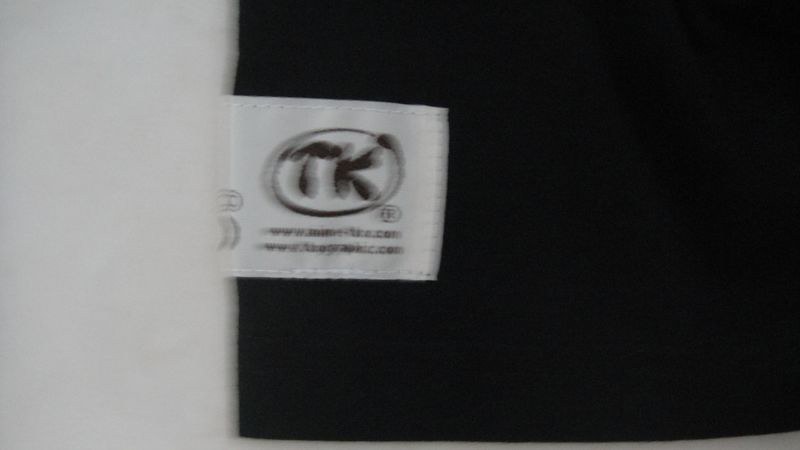The image features a black object that appears to be made of fabric, possibly a pillowcase, although the exact material is uncertain due to the texture and flow of the material that causes it to appear slightly undulating at the edges. The object is centered on a white background, providing clear contrast.

Affixed to the black fabric is a white label resembling a tag. The label prominently displays the letters "TK" in bold, black typography inside a circular border. Adjacent to this label is the trademark symbol, "Ⓡ". Below "TK," there are multiple lines of text that end in ".com". The text likely includes "www," but the details are indiscernible because the writing is too blurry to make out clearly.

Despite the artifact's indistinct shape and ambiguous material properties, the white label stands out sharply against the dark fabric, making the printed information partially legible.